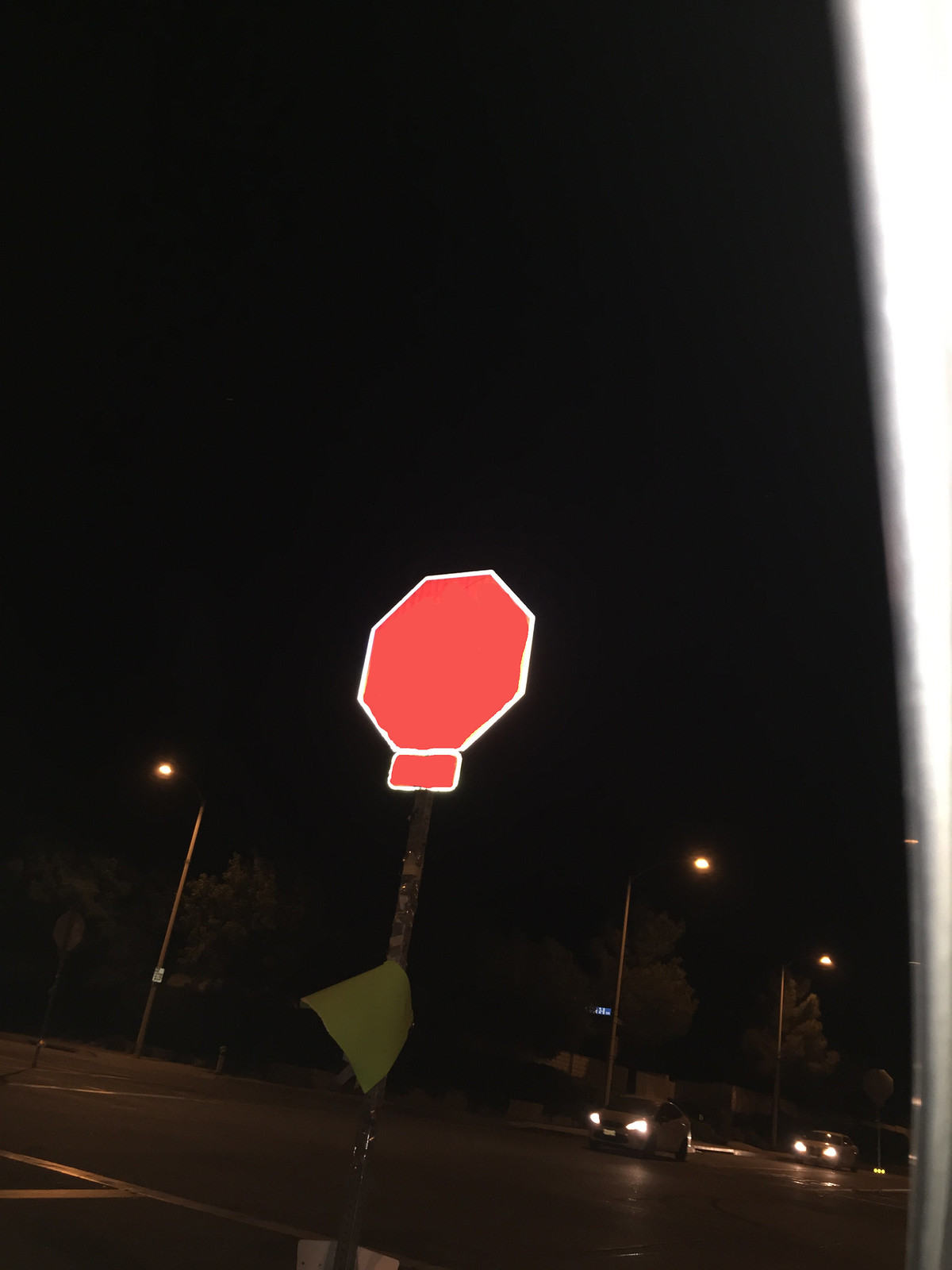The image depicts a nighttime urban scene dominated by a jet-black sky and a meticulously detailed intersection. At the forefront stands a prominent red octagonal stop sign, missing its usual "STOP" lettering, perhaps due to vandalism. The sign, outlined in white, is mounted on a black metal pole and appears to have a dark green paper partially attached to it, fluttering in the wind. The street features a yellow line down the middle, illuminated by the headlights of several cars driving along the road. Tall streetlights on metal posts line both sides of the street, casting their glow on the surroundings, including the silhouetted trees and faint outlines of walls. Additional stop signs and streetlights can be seen in the distance, reinforcing the sense of a busy, well-lit intersection at night.